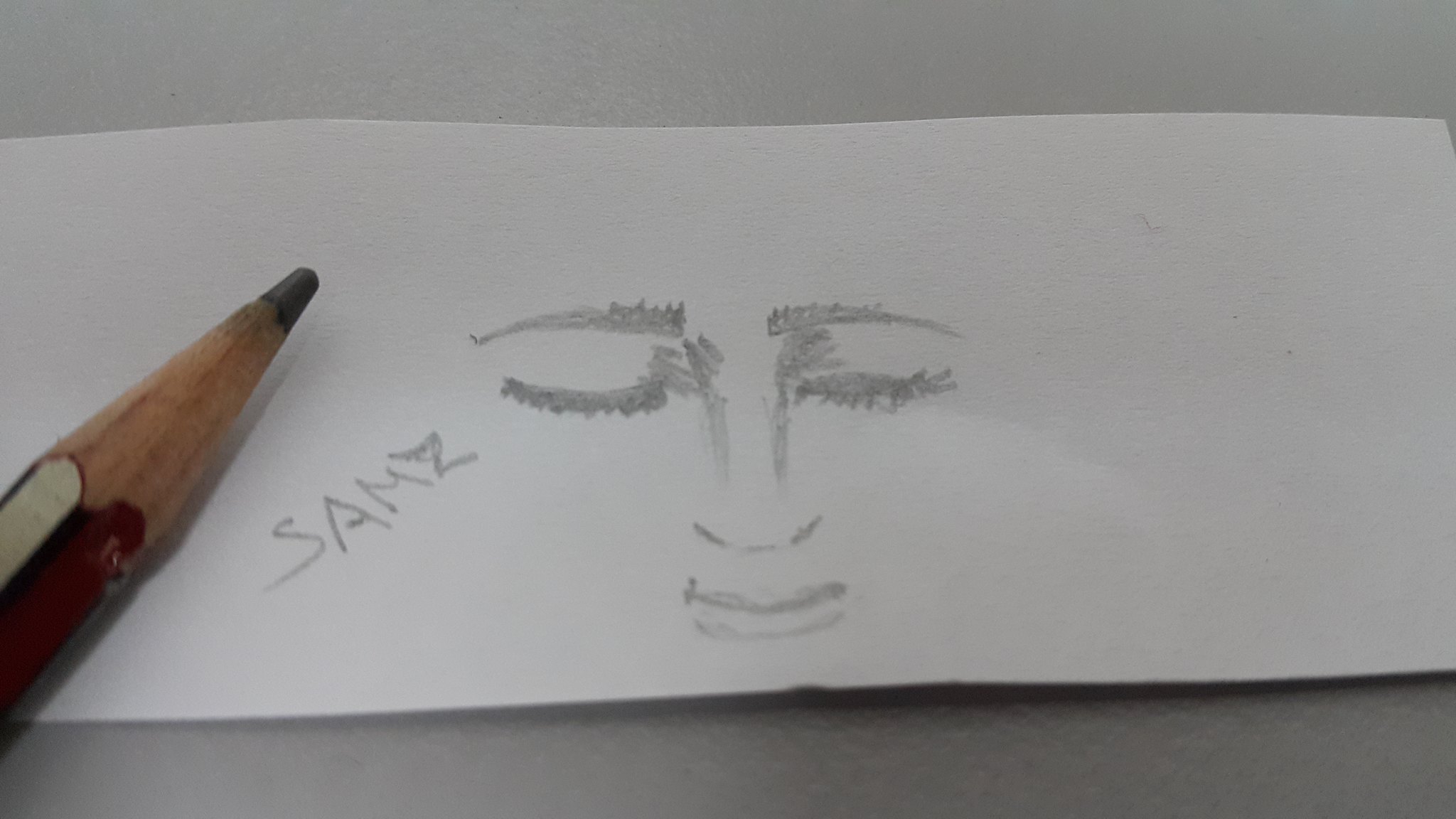This is a detailed landscape-format photograph showcasing a high-end, rectangular sheet of textured paper, which is whiter than the surface it rests upon, possibly a white or gray table. The sheet features a light, delicate sketch of a human face, most likely of a woman with her eyes shut, suggesting she might be sleeping. Key facial elements like the eyebrows, nose, bottom of the eyelashes, and lips are clearly depicted, even without additional facial outlines like cheeks or ear shapes. To the left of the face, the name "SAMS" is inscribed in capital letters. Also on the left side, the partial tip of the red-and-white pencil used for the drawing, with a light brown portion near the top and a dark black tip, is visible. The entire sketch is rendered in black pencil, centrally located against the pristine, high-quality paper, emphasizing the simple yet evocative artistry.